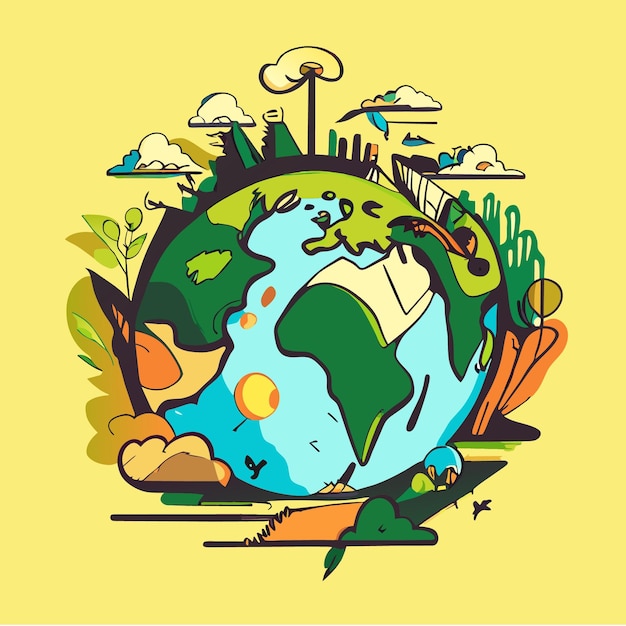The image is a playful, cartoonish illustration of the Earth as seen from the perspective over Africa, rendered against a bright yellow background with orange accents. The landmasses are colored in green and blue, with Africa prominently visible, and sections of the Middle East, North America, Europe, and Asia discernible despite their lack of precise accuracy. Surrounding the globe are numerous whimsical elements, including sprigs of plants, clouds, trees, what appears to be mountain ranges, and a cityscape. Additionally, there are birds depicted in the scene, adding to the vibrant and busy visual activity. This detailed and colorful drawing, which lacks any written text or visible signatures, evokes a sense of celebration and could easily serve as a poster for an Earth Day event or a similar environmental cause.